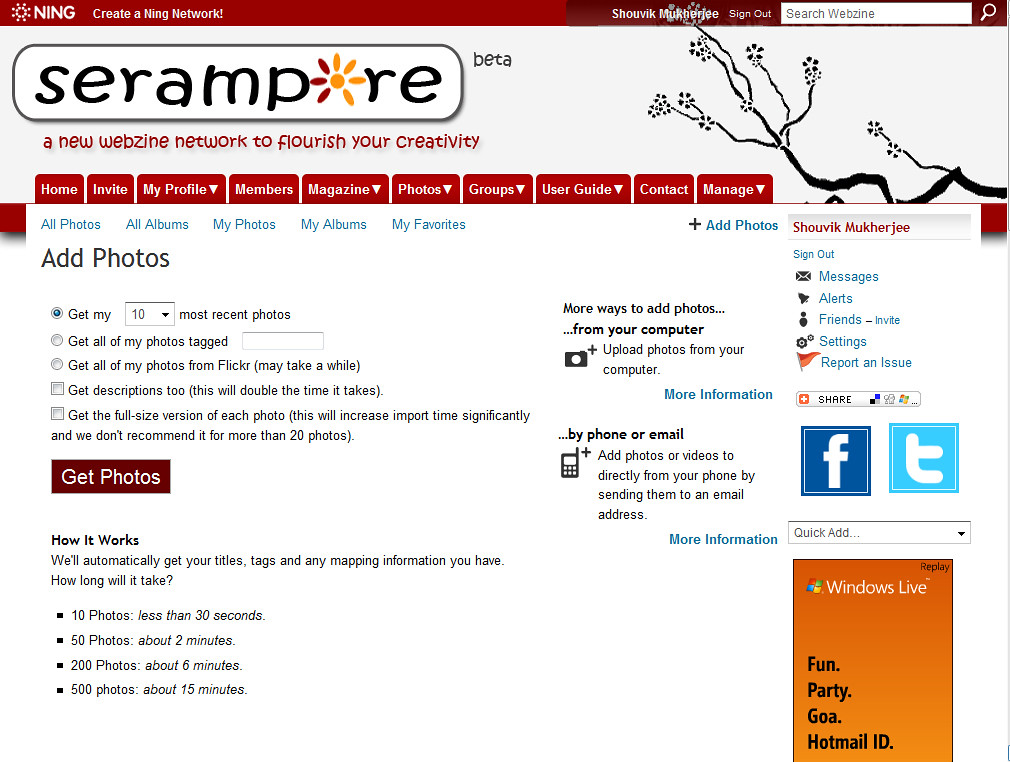This detailed screenshot depicts a white-background homepage of a website featuring intricate red borders and a header with a maroon strip at the top. On the top left, the logo reads "NING," with the tagline "Create a Ning Network." Towards the top right, it displays the account holder's name "Shobit Mukherjee," a sign-out option, and a search bar labeled "Search Webzine."

Below this header, a prominent logo reads "Serampore Beta," with the tagline "New Webzine Network to Flourish Your Creativity." The "O" in "Serampore" is creatively designed as a flower, while to the right of this text, there is an artistic drawing of tree branches with blooming flowers. 

Underneath, there is a primary navigation bar featuring red buttons labeled Home, Invite, My Profile, Members, Magazine, Photos, Groups, User Guide, Contact, and Manage. Each button includes a dropdown arrow for additional options. The active section is Photos, which presents further navigation options: All Photos, All Albums, My Photos, My Albums, My Favorites.

In the Photos section, detailed options for adding photos are visible. The selected option is "Get My 10 Most Recent Photos," with additional options for retrieving all tagged photos, importing from Flickr, getting descriptions, and importing full-size versions. There is also a detailed explanation of import times for different quantities of photos.

On the right side, there are icons for social interactions, including a plus symbol for adding photos, a message icon, an alerts icon, friends' invitations, settings, and a flag icon for reporting issues. Social media icons for Facebook and Twitter are present, as well as a search bar and a Windows Live advertisement with a "Replay Fun Party Goa Hotmail ID" logo.

At the bottom right, under "More ways to add photos," options include uploading from a computer or phone, with corresponding icons and more information links. The left side features a "Get Photos" button and text explaining the photo import process, detailing the approximate times required for importing varying numbers of photos.

Overall, the design emphasizes user engagement through detailed menu options, interactive buttons, social media integration, and explicit instructions for photo management.